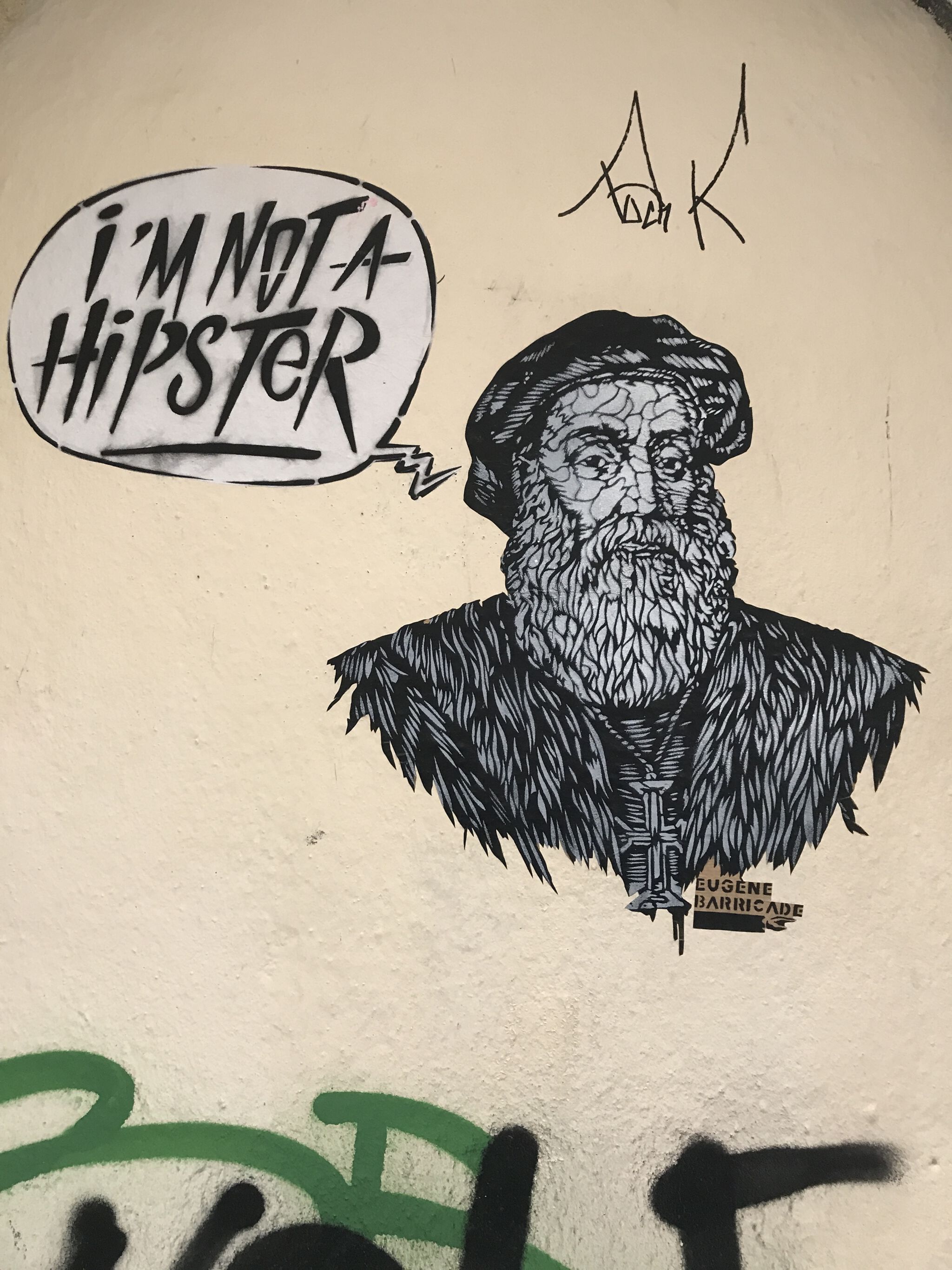The image showcases an intricate piece of street art on a light tan wall, with a strip of green and black graffiti at the bottom. The central focus is a detailed stencil or mural sticker of an elderly, bearded man, adorned in a fluffy cape and an old-style English hat, indicative of a bishop or an aristocrat. This figure is very textured, with harsh lines emphasizing the cracks on his stern face, giving the appearance that he’s been chipped into pieces but remains whole. Around his neck hangs a prominent cross. A brown sign beneath him is labeled "Eugene Barricade," though it's unclear if this refers to the subject or the artist. Adding to the artwork’s whimsy, a thought bubble emanates from the man's head in flamboyant, albeit jagged, lettering that proclaims, "I'm not a hipster," with 'hipster' notably underlined. Above the main artwork, there’s a curious addition of marker graffiti that spells out "R-O-C-K." The entirety of the man's depiction is rendered in stark monochrome, contrasting with the vivid graffiti below.